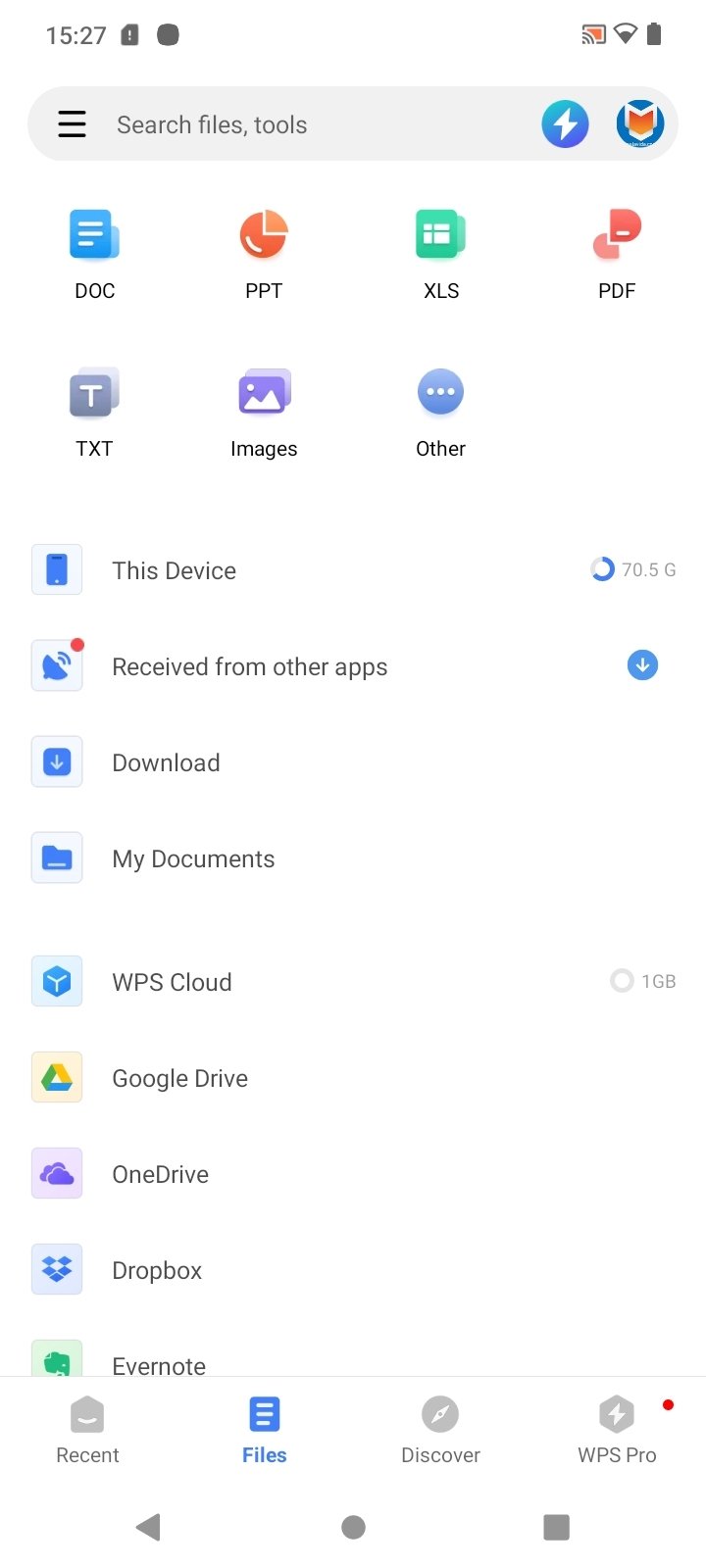This screenshot captures the interface of a file management application on a device. The interface showcases various options for file locations, including ".pdf," ".xl," "images," and ".txt." These options are categorized under different sections such as "Received from Others," "Downloads," "My Document," "WPS Cloud," "Google Drive," "OneDrive," "Dropbox," "Evernote," "Recent," "Files," and "Discover."

Visible on the interface are several icons corresponding to these categories, as well as icons for battery status, file search, and tools. The device indicates that it has a total storage capacity of 70.5 GB. A notable element is the red dot appearing next to "Received from Other Apps," which might denote notifications or new files. Additionally, "WPS Cloud" shows a storage usage of 1 GB. The text for each category is presented in black and gray, enhancing readability and visual distinction.